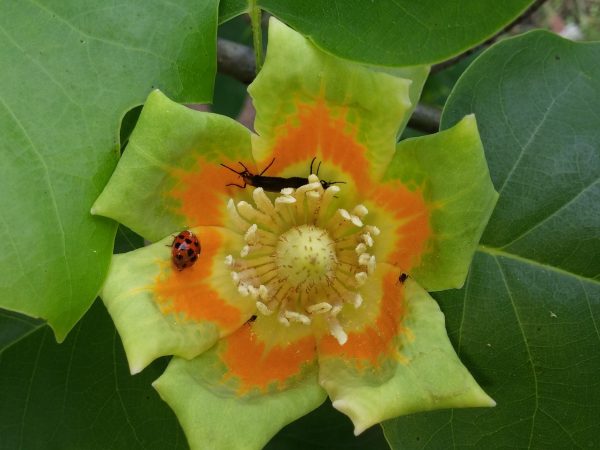The image is a close-up photograph of a tulip tree flower at its core. The flower's central part features light green with white pistils extending outward, creating a prickly texture. Surrounding this core is a star-shaped yellow area, which gradually transitions to an orange ring. The flower is encased by light green petals that form a six-petal structure. Notably, on the left side of the flower, a red ladybug with black spots is visible. Above the ladybug, a longer, small black insect, resembling a cricket, is resting on one of the petals. The entire flower is framed by large, dark green leaves with prominent veins, surrounding it from all directions—left, right, top, and bottom. The image, taken during daylight, is detailed enough to show additional small spots, possibly more tiny insects, scattered across the petals. The combination of vibrant colors and the presence of insects makes for an appealing and intricate photograph.